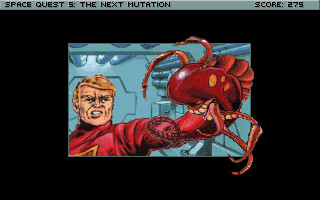A captivating screen capture from the classic video game "Space Quest V: The Next Mutation." In this image, the game title is prominently displayed in the top left corner, while the score, a solid 275, is shown on the top right, providing context that this is a still from an old video game. The background is predominantly black, enhancing the focus on the central characters. At the center, a superhero-esque figure clad in a striking red outfit with distinctive yellow lettering stands with a triumphant, somewhat menacing expression. His stance exudes confidence as he holds up a mutated alien creature, also dressed in red. The scene captures a moment of victory and intensity, drawing viewers into the nostalgic ambiance of the game.